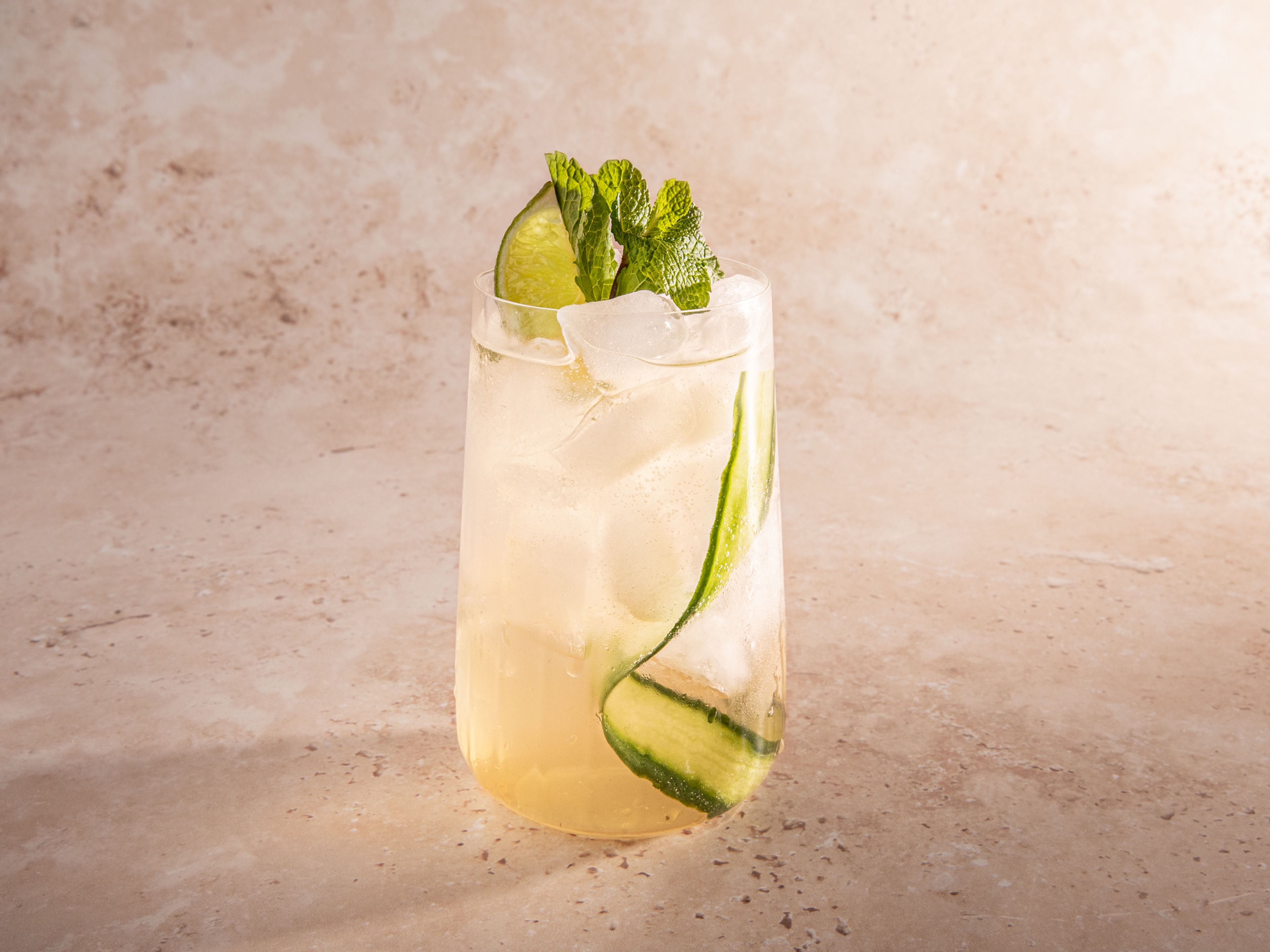This portrait photo captures a glass, centrally placed against a light tan, marble-like backdrop. The glass contains what appears to be a mojito, showcasing a light golden, fizzy liquid. Topping the drink, a lime wedge juts out to the left, complemented by a sprig of mint in the center. Inside the glass, ice cubes glisten alongside a flat, whole slice of cucumber on the right. The overall color palette is a harmonious blend of pinkish-brown, white, and green, accentuating the refreshing and inviting nature of the beverage.